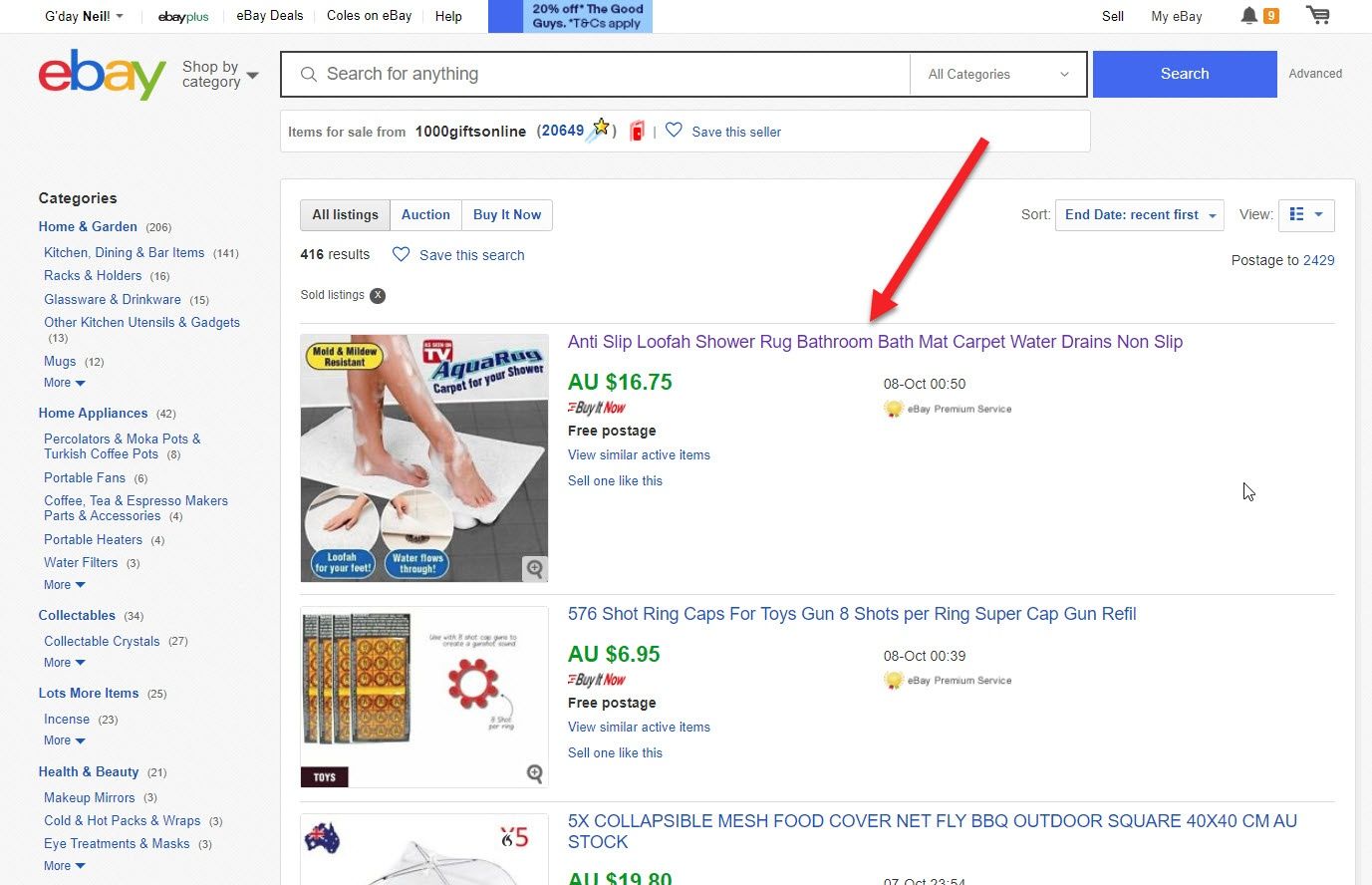The image depicts the eBay website interface. In the upper left corner, the familiar eBay logo is displayed. Following the logo, the top navigation menu lists several options: the username "G-Day Nail," indicating the user is logged in, and options for "eBay Plus," "eBay Deals," "Golds on eBay," and "Help."

Prominently highlighted in the center of the page is a red arrow pointing to a specific product listing among three items. The highlighted product is described as an "anti-slip loofah shower rug, bathroom bath mat, carpet, water drains, non-slip." The price for the item is AU $16.75. Below the price, there is a "Buy Now" button, and it mentions "Free postage." Additionally, there's an option to "View Similar Active Items" and a prompt to "Sell one like this." An image of the mat is displayed to the left of the description, showcasing its appearance.